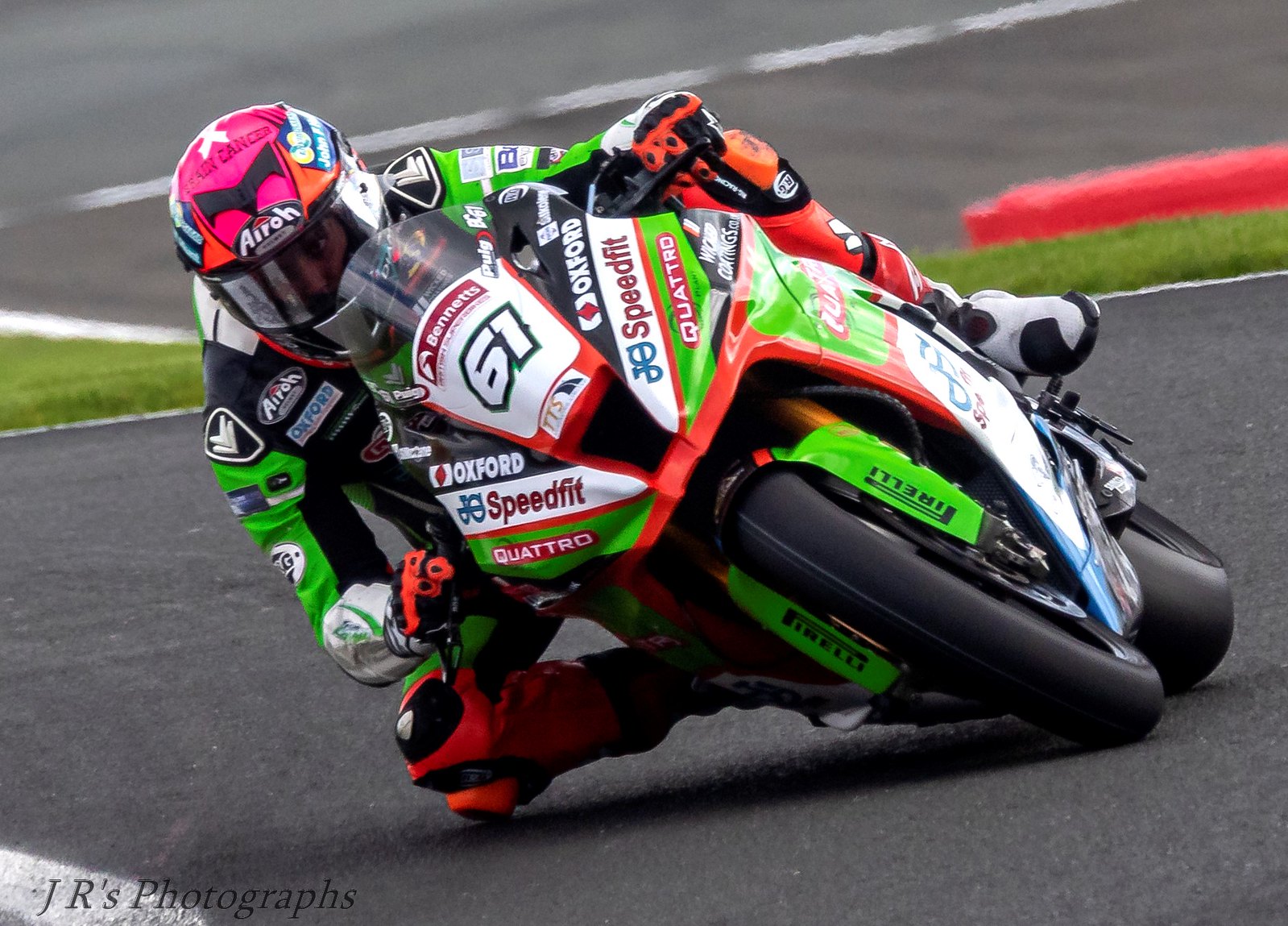The image showcases a motorcycle rider in a high-speed race, captured mid-turn with his bike angled sharply to his right, nearly scraping the ground. The rider's body leans dramatically to the left from our perspective. His bike is predominantly green with orange and white accents, adorned with various sponsor logos including "Bennett's" on a red banner above the number "61" on a front protective plate. The sides feature "Oxford" and "Speedfit" on black and white strips respectively, and a green strip at the bottom displays "Quattro". The wheel bears the lettering "PIRELLI". The rider is clad in a matching outfit with prominent green and orange elements, and his helmet stands out with a large pink section labeled "Airo" above the visor. In the bottom right corner of the image, the photographer's credit reads "JR's Photography" with the initials and the P capitalized.